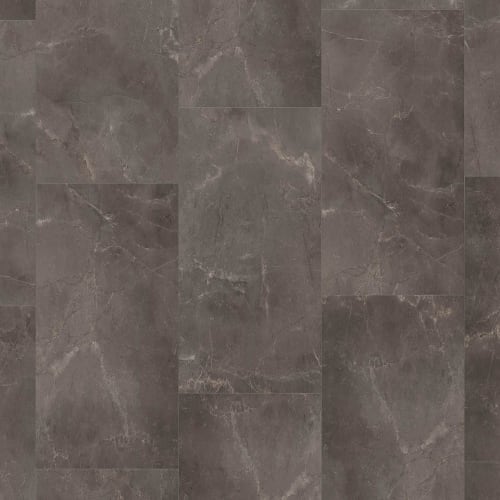This image shows a tiled surface with rectangular stone tiles arranged in a staggered masonry pattern, similar to a brick wall. The tiles, which are taller than they are wide, feature varying shades of gray from medium to dark, interspersed with lighter gray veining. These veins create a subtle, smoke-like effect within the stone. The seams between the tiles are not aligned vertically, enhancing the staggered design. The exact application of this tiling is unclear, but it could be used for flooring or a wall, possibly in a bathroom or as a countertop backsplash. The lighting is even, revealing no shadows, and highlighting the natural texture and detailing of the stone tiles.